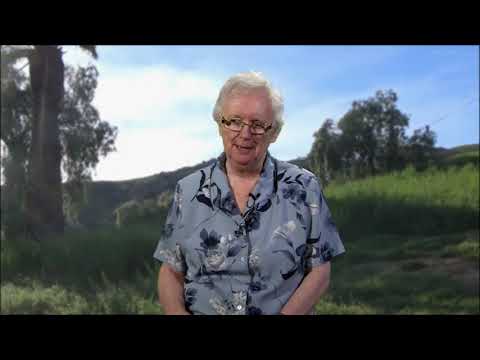An older person with short white hair and glasses sits centrally against a seemingly artificial backdrop. The person is wearing a gray, short-sleeve button-up Hawaiian shirt adorned with black and white flowers. In the background, which appears to be either a green screen or a fabric backdrop, there is a scenic depiction of a grassy field with a large tree to the left, additional trees in the rear, and a clear blue sky with a few clouds suggesting late afternoon. The lighting discrepancies hint at the background being digitally or manually generated, as the person is fully lit with distinct shadowing incongruent with the backdrop's natural elements. The attire and setting give an impression of a casual, perhaps staged, environment akin to a studio interview or presentation.